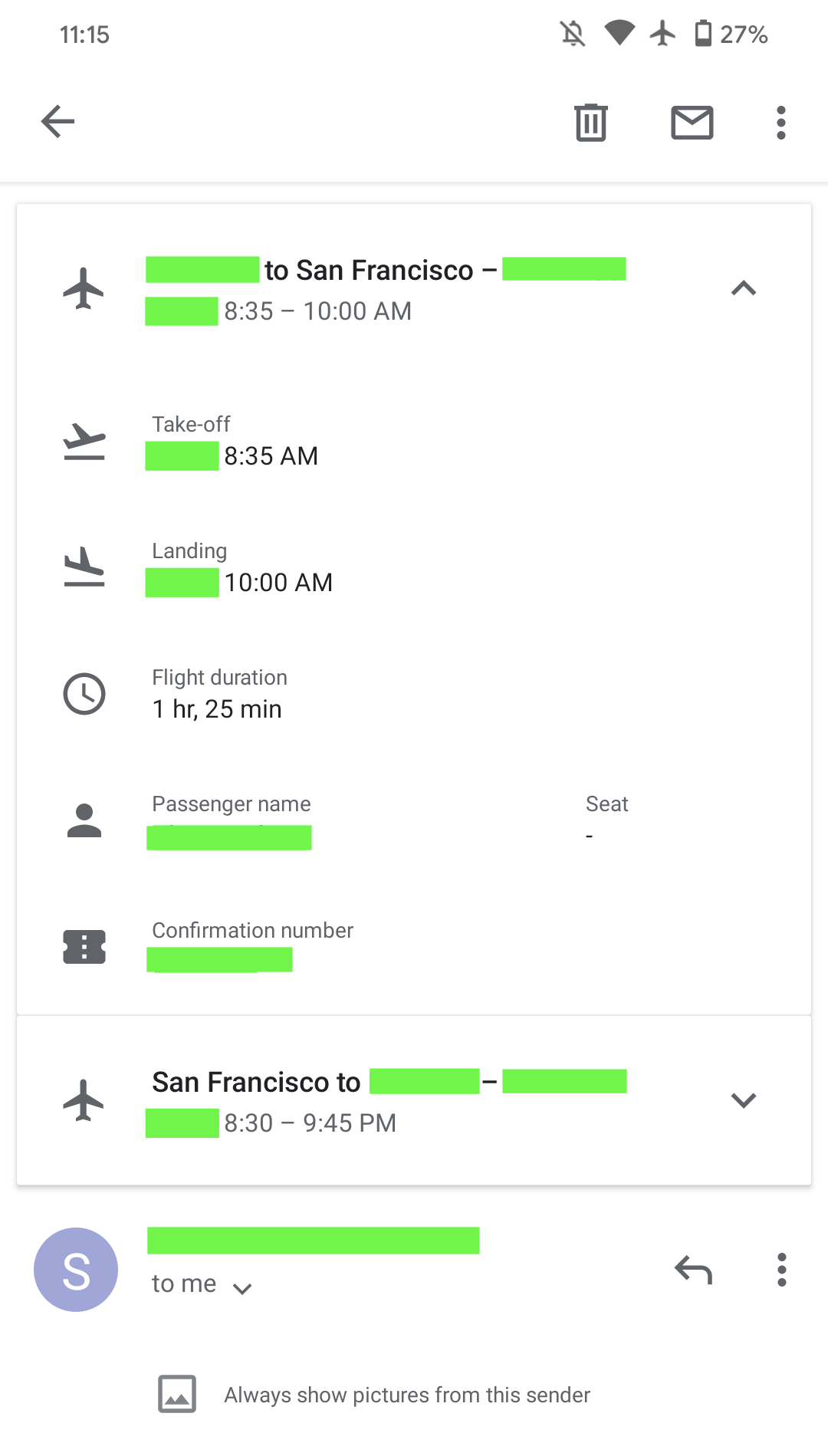The image shows a smartphone screenshot displaying detailed flight information, partially obscured by neon green highlights. This highlights some key details such as the destination airport, passenger name, and other personal information. The visible segments indicate a flight from San Francisco, with the city name appearing twice on the screen.

The flight is scheduled to take off at 8:35 a.m. and land at 10:00 a.m., with an overall duration of 1 hour and 25 minutes. Under the passenger section, the seat number is represented by a dash, signifying no specific seat assignment, and the information number is also obscured by the green highlight.

At the bottom of the screenshot, there is mention of a return flight from San Francisco to the covered destination, scheduled to depart at 8:30 p.m. and arrive at 9:45 p.m. The format of the text and layout suggests that this information is embedded within an email or a messaging application. Additionally, on the left side of the "to me" section, there is an avatar featuring a white "S" inside a lavender circle.